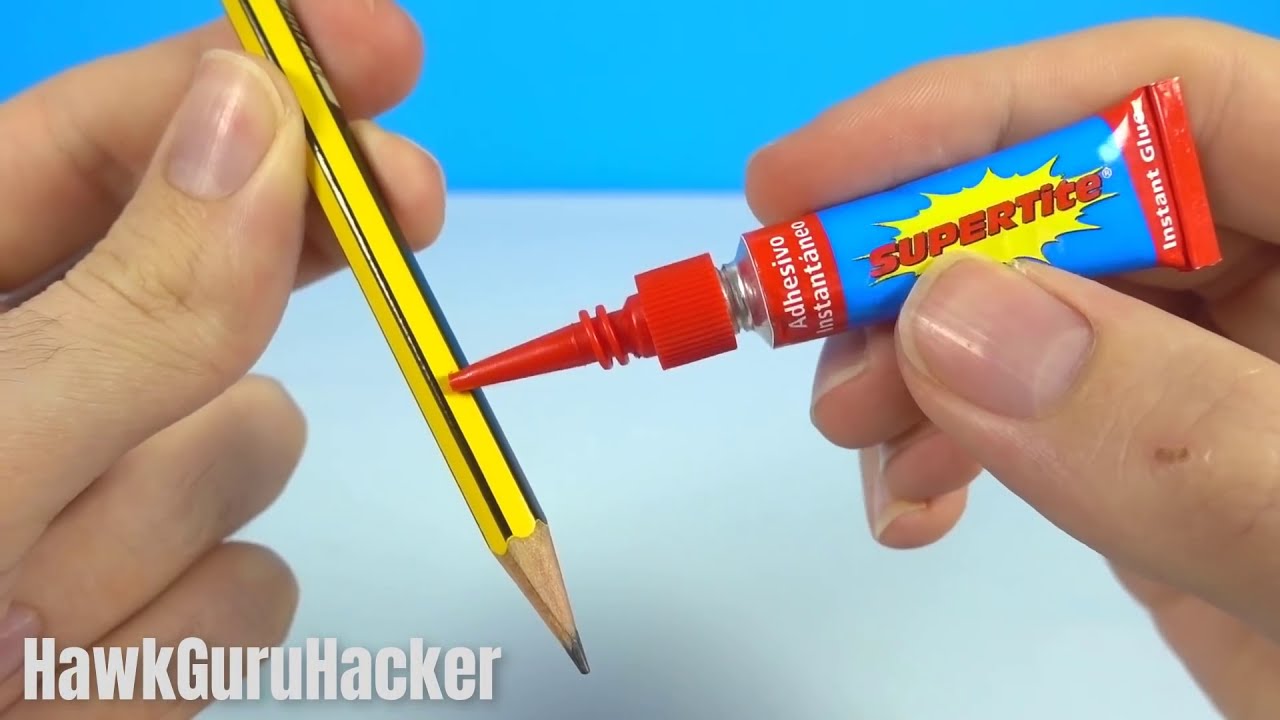In vivid detail, the image shows a light-skinned male's two hands against a background that transitions from a dark blue at the top to a lighter shade below. The left hand, displaying slightly folded ring and pinky fingers, grasps a yellow pencil with two black stripes along its length and a sharpened point. A clear view of the thumb's fingernail is visible. In the right hand, the man holds a tube of super glue, identified as "Super Tight" in red font prominently displayed within a yellow, superhero-like burst design on a blue label. The tube features a gray section and a red tip. Notably, the thumb has a small scab. The glue is being applied to the pencil tip. In the lower left corner, the words "HAWK GURU HACKER" are written in white, capital letters, emphasizing a potential DIY or instructional context.